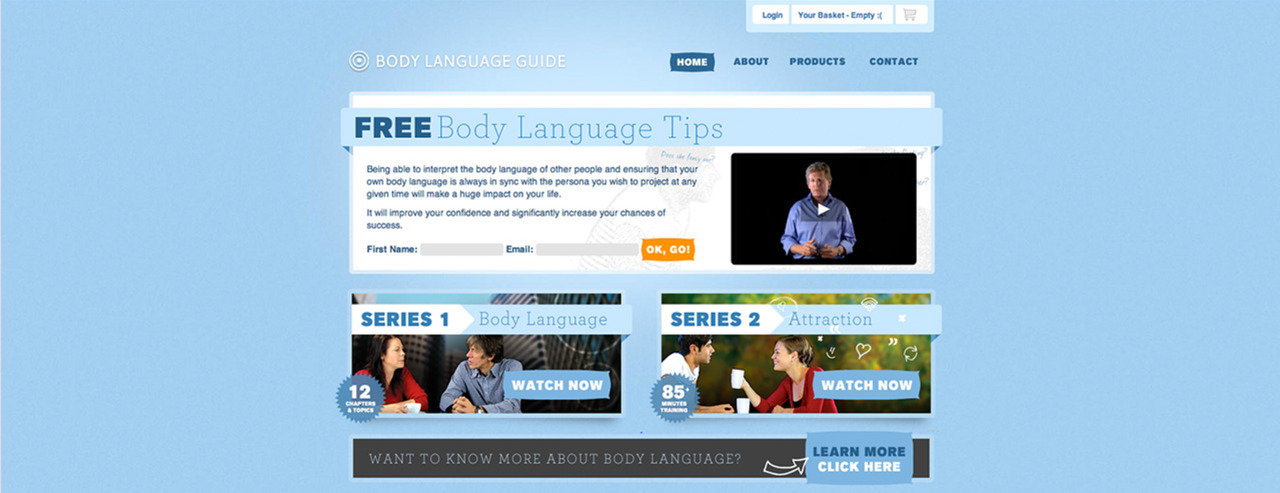Screenshot of the "Body Language Guide" website homepage, featuring a prominent name and logo at the top left. To the right, the main navigation menu includes links to Home, About, Products, and Contact, alongside a login button at the top right. The homepage is highlighted in the navigation menu, indicating the current page view.

The central section of the homepage showcases a bold banner reading "Free Body Language Tips," accompanied by a brief introductory text and a form for users to enter their name and email address. To the right of this form, there is a small embedded video providing additional information.

Below the main section, two smaller squares contain images with titles: "Series 1: Body Language" and "Series 2: Attraction," each accompanied by a "Watch Now" button, inviting visitors to explore video content on these topics.

The final section at the bottom of the page is a gray rectangle with a call-to-action: "Want to Know More About Body Language?" An arrow points to a large blue button labeled "Learn More, Click Here," likely leading to more in-depth resources.

The website's design features a clean, light aesthetic, dominated by baby blue, white, and gray hues, creating an inviting and easy-to-navigate interface.